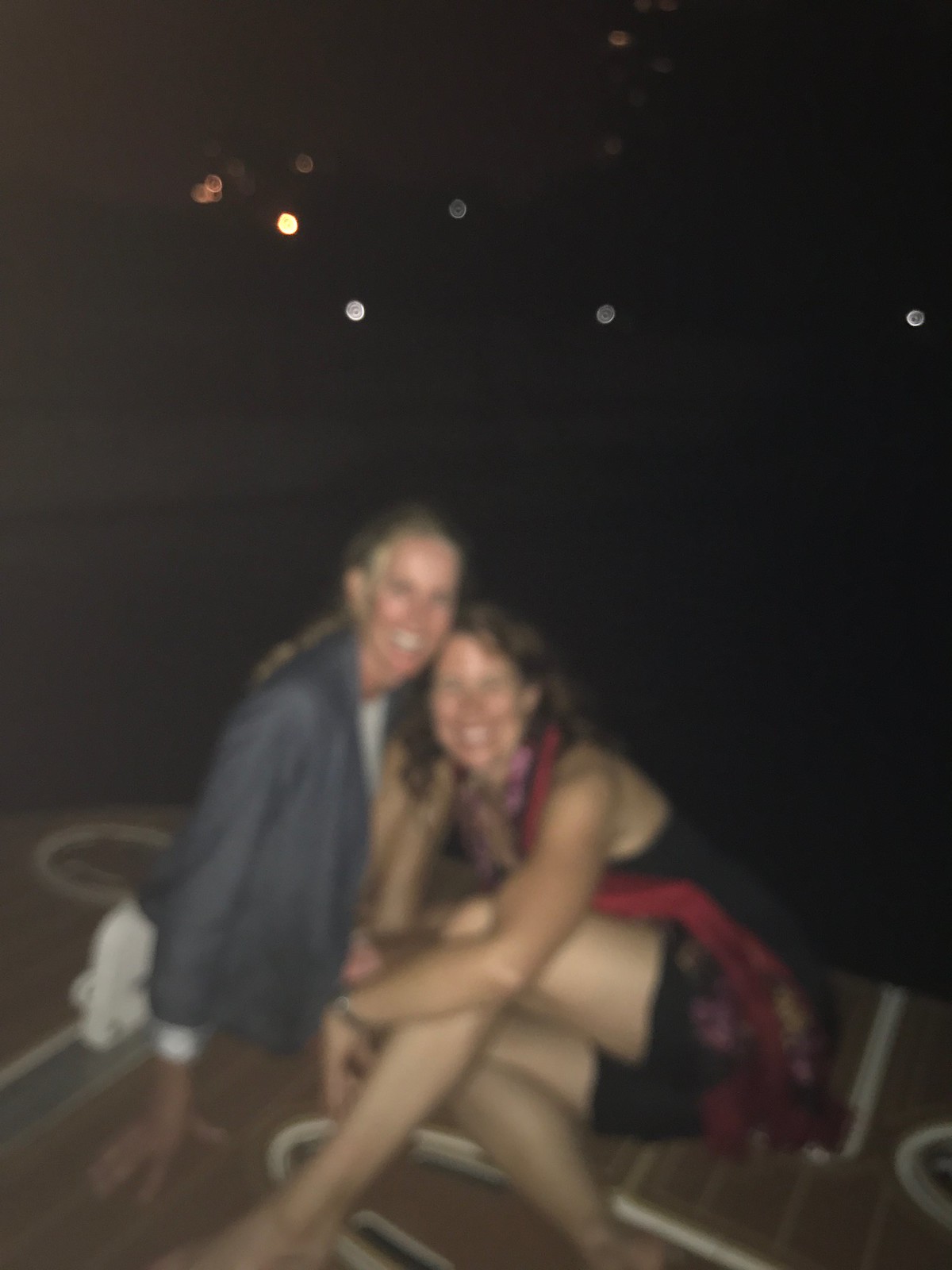In this nighttime amateur photograph, two girls who appear to share a close, possibly familial, bond are seated on what seems to be the stern of a boat. The older girl, positioned on the left, wears a pair of shorts, hinting at a summertime setting, and is also clad in a long-sleeve jacket, suggesting a comfortable, casual outing. Despite the blurry quality that makes distinguishing precise details difficult, their faces and bodies reflect the use of a flash in low-light conditions. The backdrop is a deep, enveloping black, punctuated only by distant lights that create a bokeh effect, adding a touch of whimsy to the otherwise dark scene. No text accompanies the image, leaving the focus solely on the subjects and the serene, nocturnal ambiance.